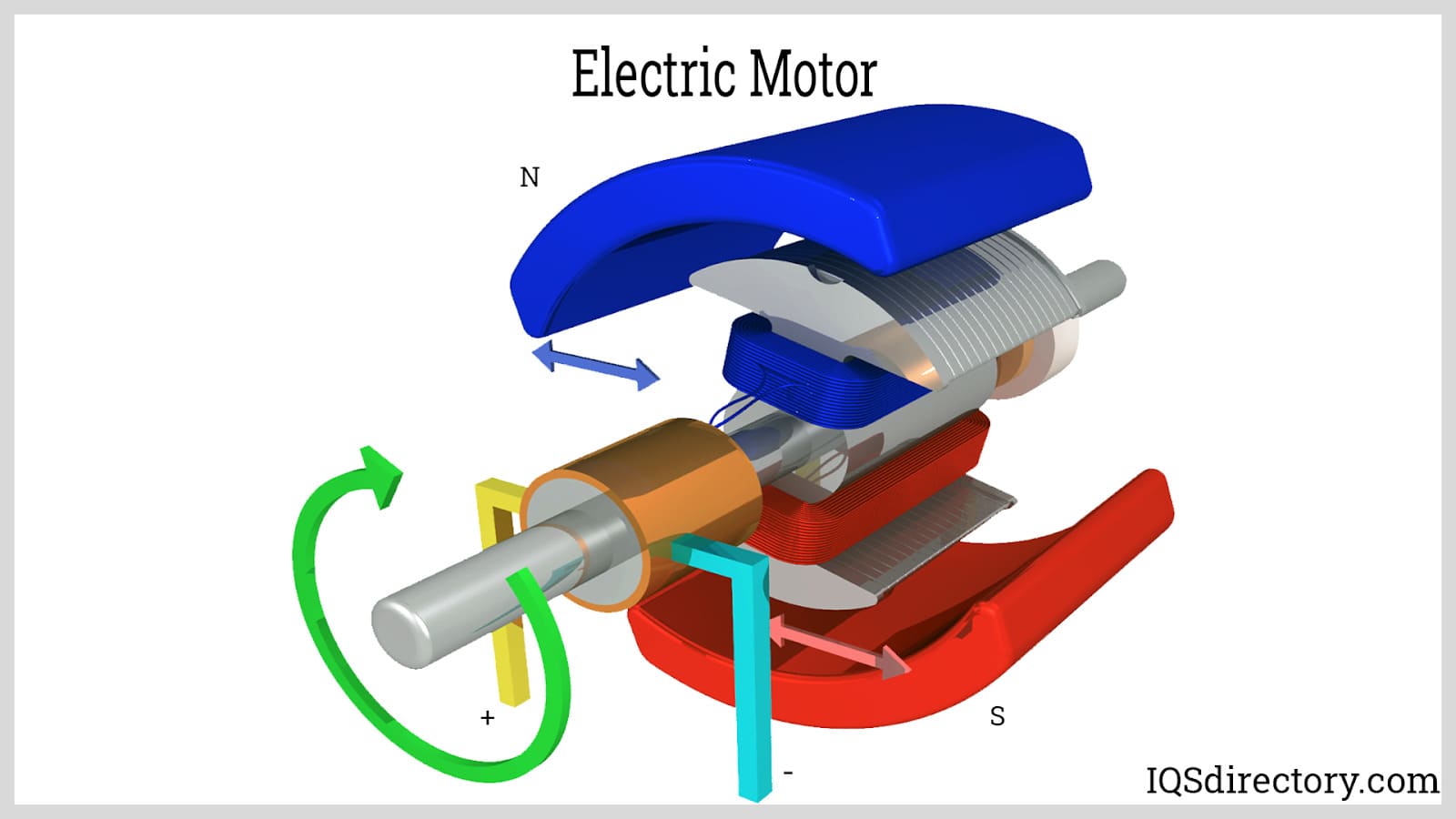This detailed, computer-generated image illustrates the inner workings of an electric motor. Displayed prominently at the top, the caption "Electric Motor" is written in black. The motor's components are separated to reveal their intricate details, with vivid colors guiding the viewer through its structure. A blue piece labeled 'N' designates the North pole at the top, while a red piece labeled 'S' designates the South pole at the bottom. The metallic parts, presumably magnets, are connected to cylinders featuring blue and red components. Arrows, color-coded to indicate rotation and direction, are scattered throughout the illustration: a green arrow at the bottom left moves counterclockwise, while a blue arrow at the top and a red arrow at the bottom point to the sides. Plus and minus signs are also present, with plus on the bottom left and minus on the bottom right. The entire image is framed against a gray border, with the website iqsdirectory.com marked in black at the lower right corner. The diagram is rich in colors, featuring shades of blue, gray, copper, yellow, green, turquoise, red, and light pink, corresponding to various parts and designations within the motor. Numbers 1 to 11 are also visible, likely indicating different engine parts.